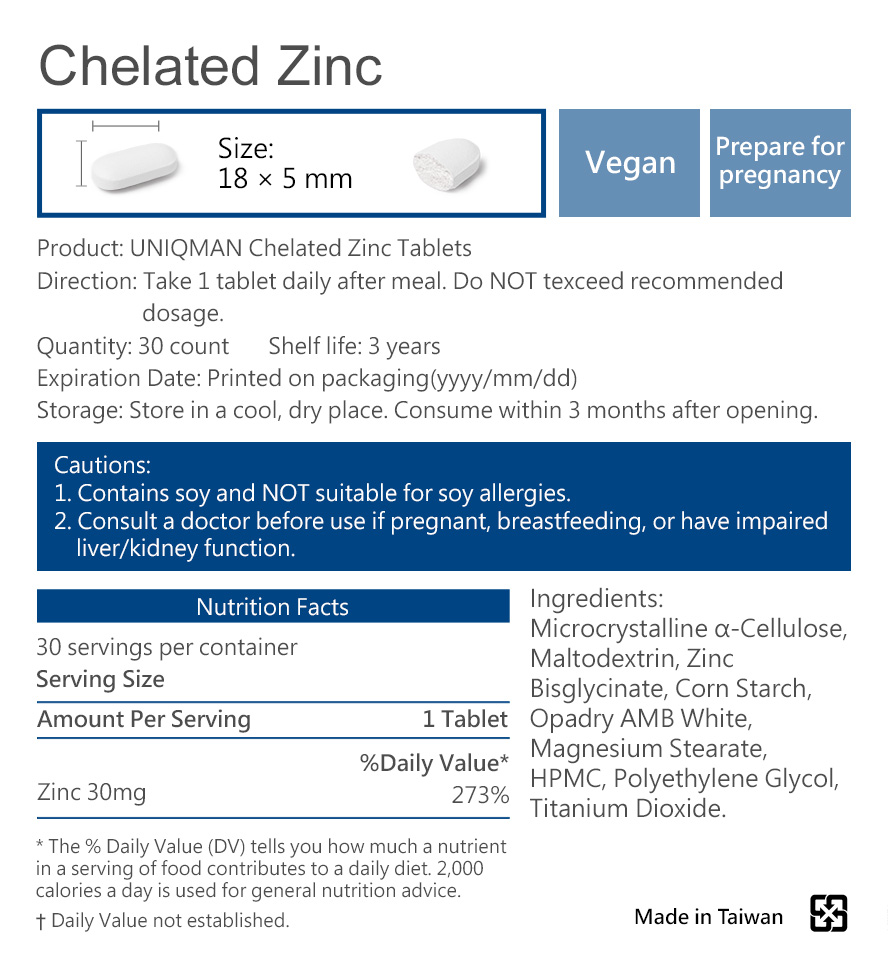This image is an informative screenshot detailing the specifications of a product called "Uni Man Chelated Zinc Tablets". At the top, the label prominently displays "Chelated Zinc". An illustration of a white pill measuring 18 by 5 millimeters is shown within a rectangle, alongside the descriptors, "Vegan" and "Prepare for Pregnancy."

Below, a detailed description follows:
- **Product**: Uni Man Chelated Zinc Tablets
- **Directions**: Take one tablet daily after a meal. Do not exceed one tablet per day.
- **Quantity**: 30 tablets
- **Shelf Life**: Three years
- **Expiration Date**: Printed on the packaging indicating year, month, and date.
- **Storage Instructions**: Keep out of direct sunlight, high temperature, and moist environments after opening. Consume as soon as possible.

A blue box labeled "Cautions" highlights:
1. Contains soy; not suitable for individuals with soy allergies.
2. Pregnant or breastfeeding women and individuals with liver or kidney disease should consult a doctor before use.

The "Nutrition Facts" section states:
- **Servings Per Container**: 30
- **Serving Size**: 1 tablet
- **Amounts Per Serving**:
  - Vitamin B1: 117% of daily value
  - Vitamin B2: 123% of daily value
  - Vitamin B6: 94% of daily value
  - Vitamin B12: 100% of daily value
  - Vitamin C: 111% of daily value
  - Niacin: 113% of daily value
  - Folate: 100% of daily value
  - Zinc: 273% of daily value

To the right, the ingredients are listed, and the bottom-right corner indicates the product is "Made in Taiwan."